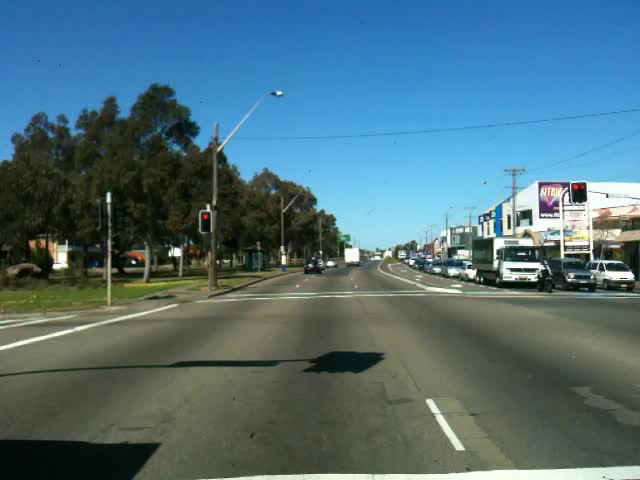In this rectangular photograph, the scene portrays a bustling suburban street under a bright blue daytime sky. The main road, which features three lanes in each direction, is heavily trafficked with an assortment of cars and trucks queued at a traffic light on the right-hand side. Leading the line of vehicles is a lone motorcyclist occupying the first lane. The left side of the image is bordered by a row of trees, providing a touch of greenery to the otherwise urban setting. Shadows cast by streetlights stretch across the scene from left to right, hinting at the sun's position in the sky. There are no pedestrians visible on the sidewalk to the left, emphasizing the dominance of vehicular activity in this suburban thoroughfare.